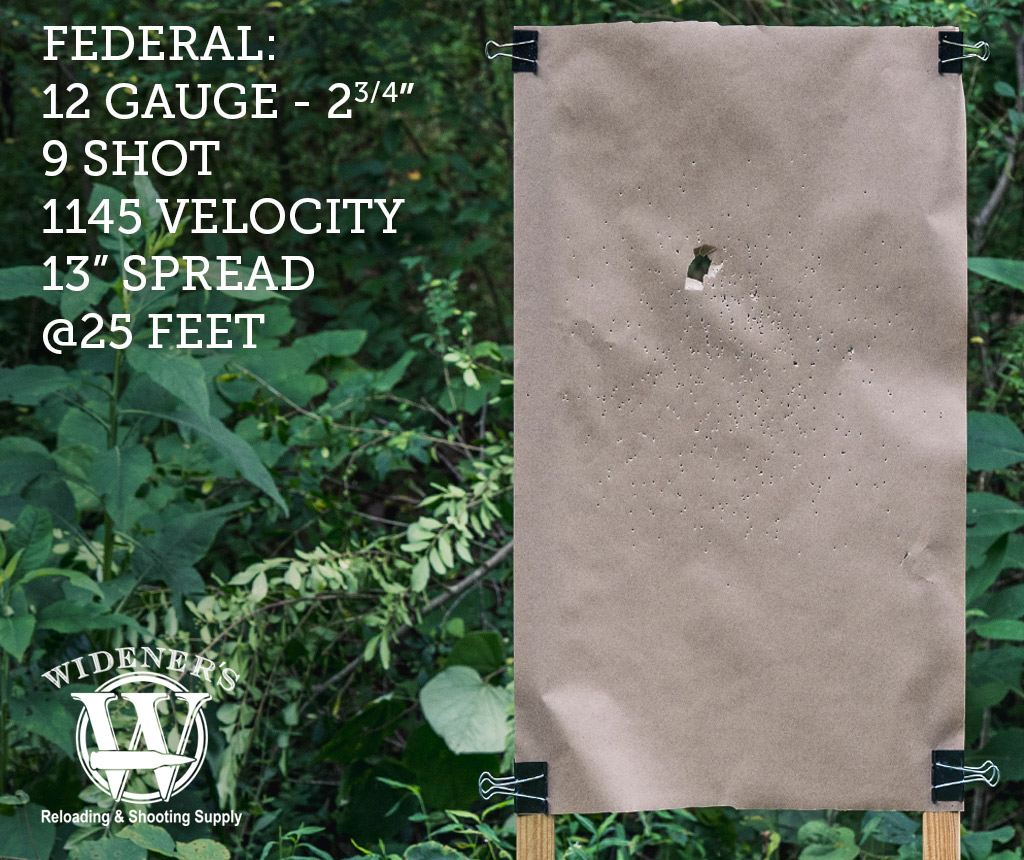This advertisement features a brown paper target held between two stakes using large paper clips, displayed against a backdrop of dense green foliage. The target bears evidence of being shot, with numerous small pellet holes and a larger central bullet hole, suggesting it was used with a shotgun. On the left side of the target, white text reads: "Federal: 12-gauge - 2 3/4 inches, 9 shot, 1,145 velocity, 13-inch spread at 25 feet." Below this, in the lower left corner, is the logo for Widener's Reloading and Shooting Supply, depicted as a "W" with a bullet running through it. This detailed scene, combining visual elements and textual information, aims to advertise the capabilities and products of the ammunition supply store.